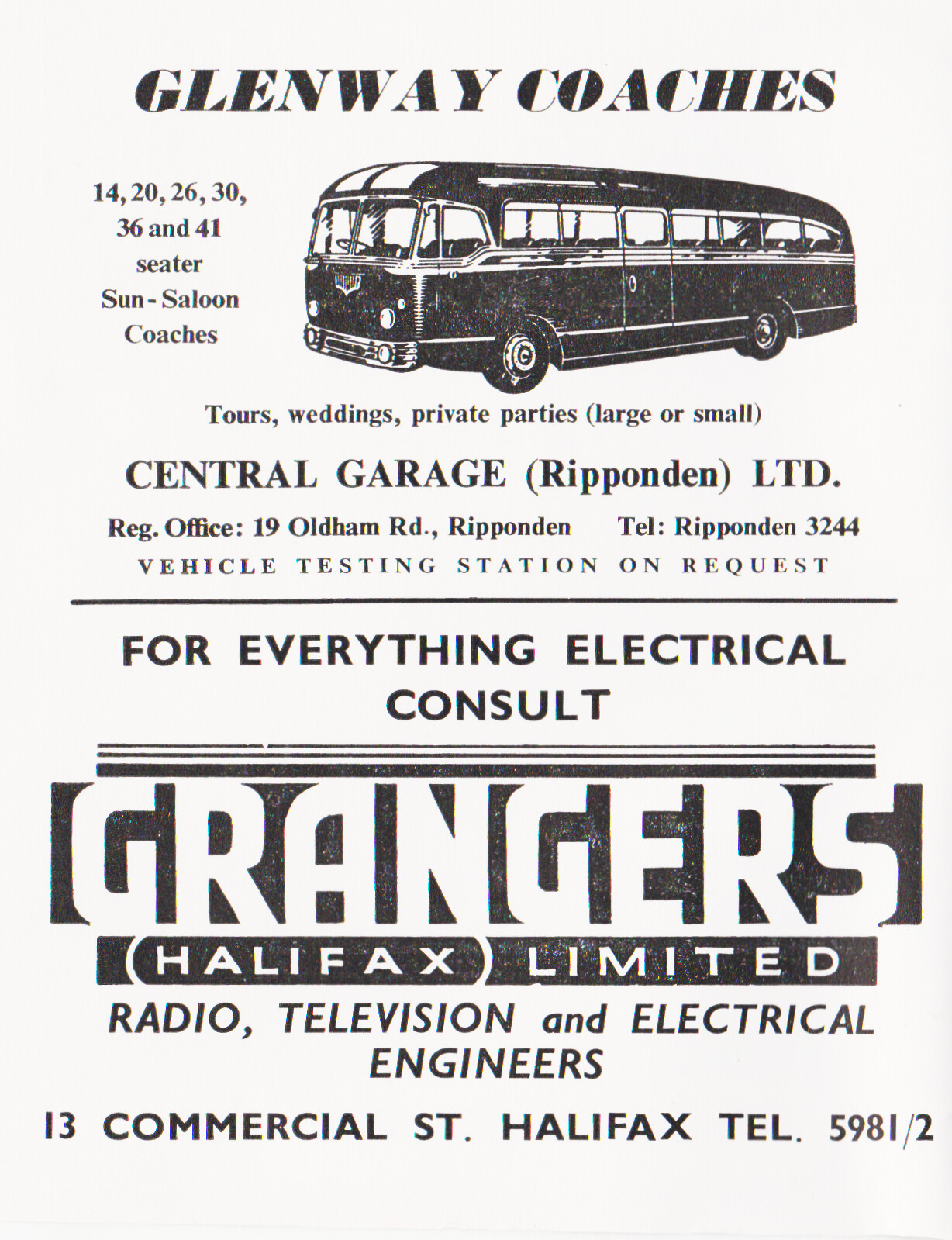This is a vintage black and white advertisement flyer. At the top, bold old-timey fonts announce "Glenway Coaches," accompanied by an illustration of a retro bus from the 1950s or 60s. To the left of the bus, "14, 20, 26, 30, 36, and 41 Cedar Sun Saloon Coaches" are listed, indicating the variety of buses available. Below the bus image, the services "Tours, Weddings, Private Parties, Large or Small" are offered. The company details are further specified with "Central Garage, Rippenden LTD, REG Office, 19 Oldham Road, Rippenden, TEL: Rippenden 3244" and a note that there is a "Vehicle Testing Station on Request."

This upper part of the flyer is separated by a black line. Below this line, the flyer transitions to a different advertisement for "Granger's Halifax Limited," specialists in "Radio, Television, and Electrical Engineers." Their contact information is provided as "13 Commercial Street, Halifax, TEL: 5981/2," indicating their location and telephone number. This suggests that the flyer may have been part of a broader publication such as a newspaper or magazine, compiling multiple business advertisements from that era.